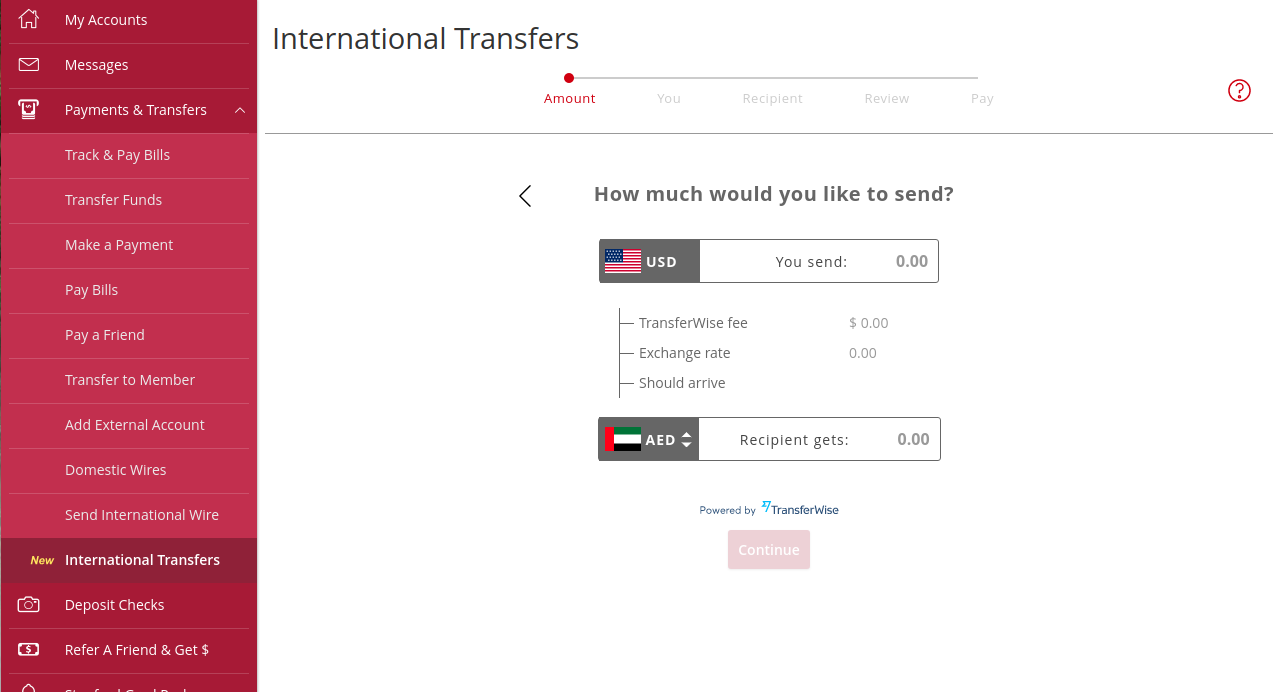This image is a screenshot of a web page from TransferWise, a service that facilitates international money transfers. The layout is divided into two main sections. On the left, a sidebar with a gradient background transitions from maroon at the top, to magenta in the middle, and back to maroon at the bottom. Written in white text, the sidebar lists various menu items including:

1. My Accounts
2. Messages
3. Payments and Transfers
4. Track and Pay Bills
5. Transfer Funds
6. Make a Payment
7. Pay Bills
8. Pay a Friend
9. Transfer to Member
10. Add External Account
11. Domestic Wires
12. Send International Wires

Highlighted among these items is "New International Transfers." Additional menu items follow, including "Deposit Checks" and "Refer a Friend and Get Money," with a corresponding dollar sign icon.

The main content area, occupying about three-quarters of the screenshot, features a white background. At the very top, the title "International Transfers" is displayed, followed by a thin line. This section appears to be the starting point for sending money internationally.

At the top of this section, it prompts the user with “Amount” and underneath it states in gray font, "How much would you like to send?" A rectangular input field follows, featuring a US flag icon and "USD" on a gray background to the left, indicating the user’s sending currency. The white portion of the rectangle is labeled "You send," where the user will input the amount they wish to transfer.

Below this input field, there are sections for additional details:
- TransferWise Fee
- Exchange Rate
- Should Arrive

Further down, another input field shows a flag icon labeled "AED" in white letters, indicating the recipient's currency. This section is labeled "Recipient gets," with a space where the received amount would be displayed after input.

At the bottom of this form, in small, faint text, the words "Powered by TransferWise" are visible. The "Continue" button at the very end appears faded, likely to become active once all necessary information is entered.